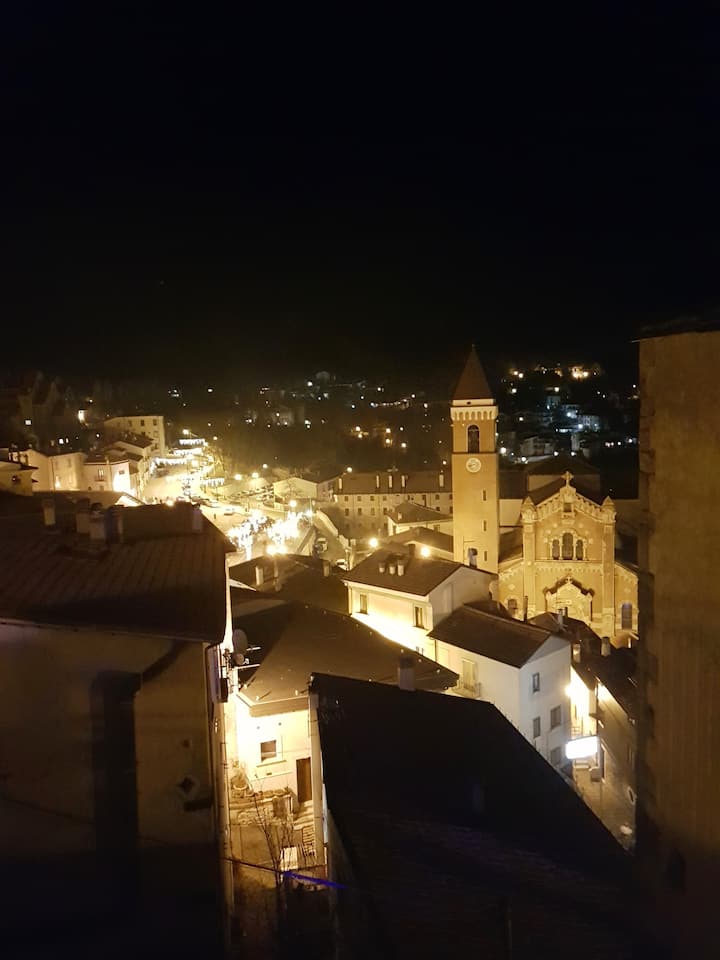The photograph captures a mesmerizing night-time view from a higher vantage point, such as a rooftop or balcony, overlooking what appears to be an old Italian town, likely Florence. The scene is bathed in a romantic, yellowish glow typical of streetlights and perhaps enhanced by a festive atmosphere. In the distance, a prominent Duomo with its large tower stands illuminated, surrounded by smaller, charming buildings. The photo also shows a bustling walking area adorned with numerous lights on the left side of the frame, contrasting with the darker regions and scattered lights of the city extending towards the hilly background. The sky above is pitch black due to light pollution, adding to the dramatic effect of the cityscape below.